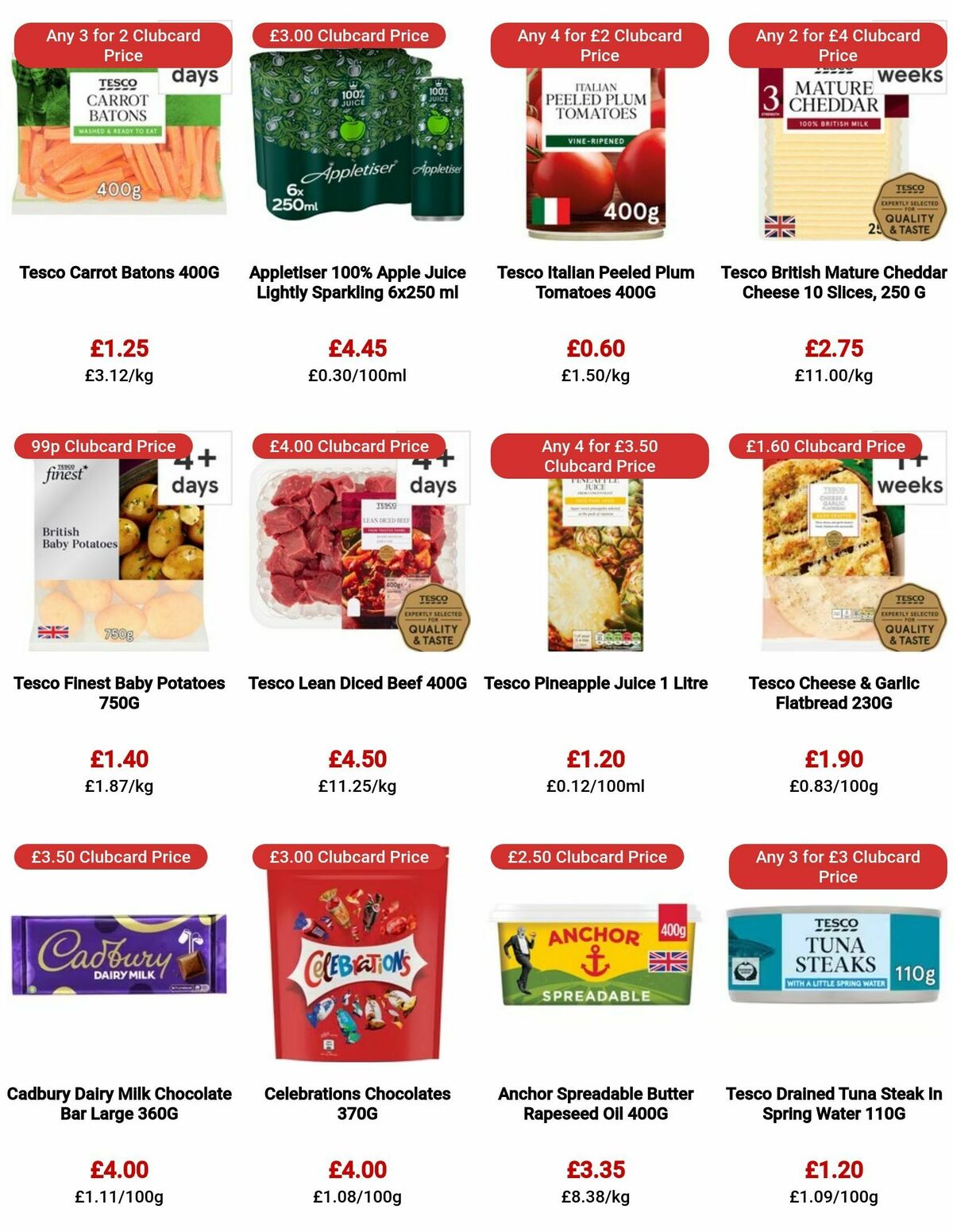A vibrant display of grocery store items showcases an array of products meticulously lined up in rows. Featured items include fresh baby carrots (400g package), sparkling apple juice (445ml), canned peeled plums, matured cheddar cheese, and baby tomatoes among other essentials like diced beef, rapeseed oil, canned tuna, and milk chocolate. Above each product, red bubble labels announce enticing club card deals, such as "Any three for two club card price." For instance, baby carrots are priced at €1.25 per 400 grams, equating to €3.12 per kilogram. Similarly, sparkling apple juice is offered at a club card price of €3, a significant discount from the standard €4.45, with detailed pricing of €0.30 per 100 milliliters. Each item's price is prominently displayed in red, alongside the unit price. The display is visually appealing with vivid photos of each product, highlighting the quantity, price, and discounts available for club card holders, all aimed at creating an informative and engaging shopping experience.